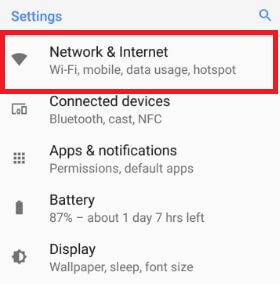The image is a screen capture of the settings application on a computing device, presented in a roughly square format with a very light gray background. At the top of the application, the word "Settings" is displayed in blue text in the upper left corner, while a blue magnifying glass icon for the search function appears in the upper right corner. 

On the main interface, there are five settings options, each accompanied by a small, simple graphic icon on the left. Both the headers, written in bold black text, and their descriptions, in gray unbolded text, are left-aligned. The first option listed is "Network & Internet," which has been highlighted with a red rectangular border. Its description reads, "Wi-Fi, mobile data usage, hotspot." Below this, in order, are the options "Connected Devices," "Apps & Notifications," "Battery," and "Display." 

The image overall is relatively small and moderately low in resolution but captures the essential layout and design of the settings application effectively.